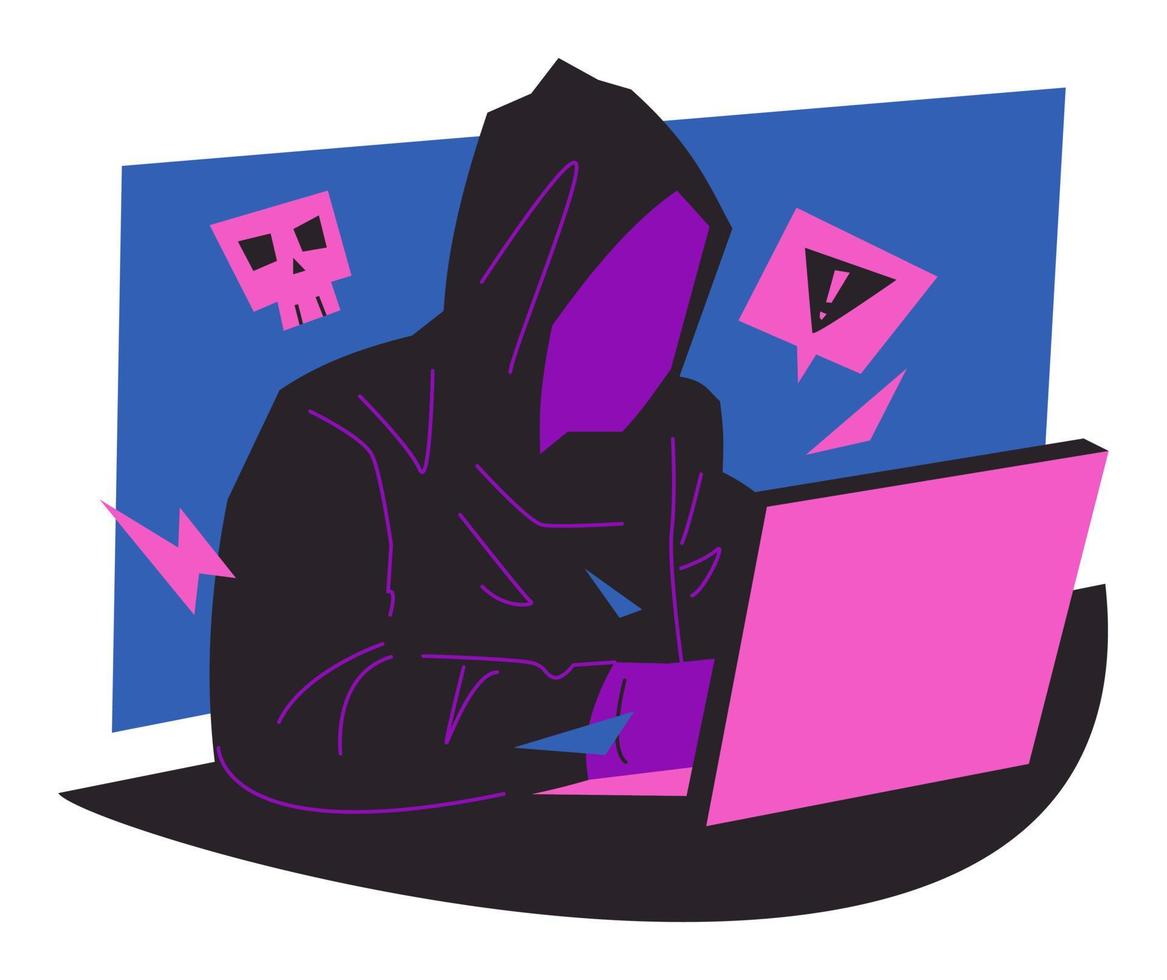The image is a stylized, possibly AI-generated or computer-drawn graphic with a corporate cartoonish aesthetic. It depicts a faceless, purple-skinned figure in a black hoodie adorned with subtle purple outlines and shadows, adding depth and shape. The figure is working intently on a hot pink laptop, seated at a black desk. The backdrop is a blue screen that provides a sense of depth to the scene. Emojis, including a skull and a warning sign, are positioned on either side of the figure, signaling a sense of urgency and suggesting nefarious activities such as hacking. The overall composition evokes a modern, somewhat ominous portrayal of a cyber hacker.